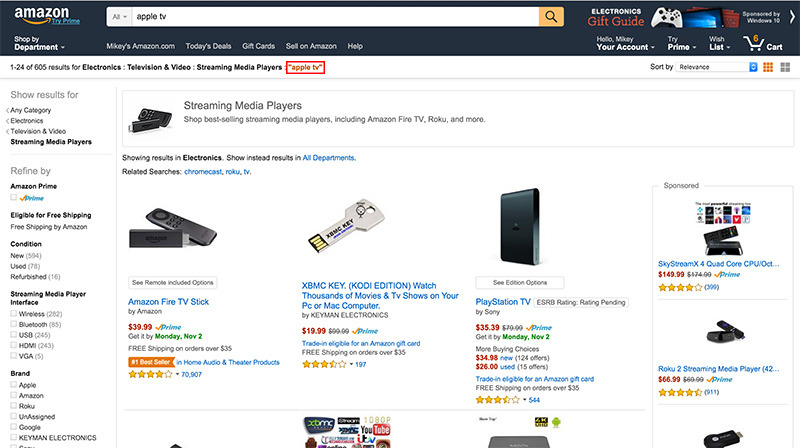A user on an Amazon website searches for "Apple TV" and is browsing the "Streaming Media Players" category. The results initially set to "Electronics" also suggest viewing results from "All Departments" with related searches including Chromecast, Roku, and TV. Featured products include:

1. **Amazon Fire Stick** - Priced at $39 with free shipping on orders over $35.
2. **XBMC Key** - Offers access to thousands of movies and TV shows on PC or Mac for $19.99.
3. **PlayStation** - Multiple pricing options available at $35, $39, $34.98, and $26.
4. **SkyStream X Quad-Core** - Priced at $149.99.
5. **Roku Streaming Media Player** - Available for $66.99.

Further details of additional products were not fully visible.